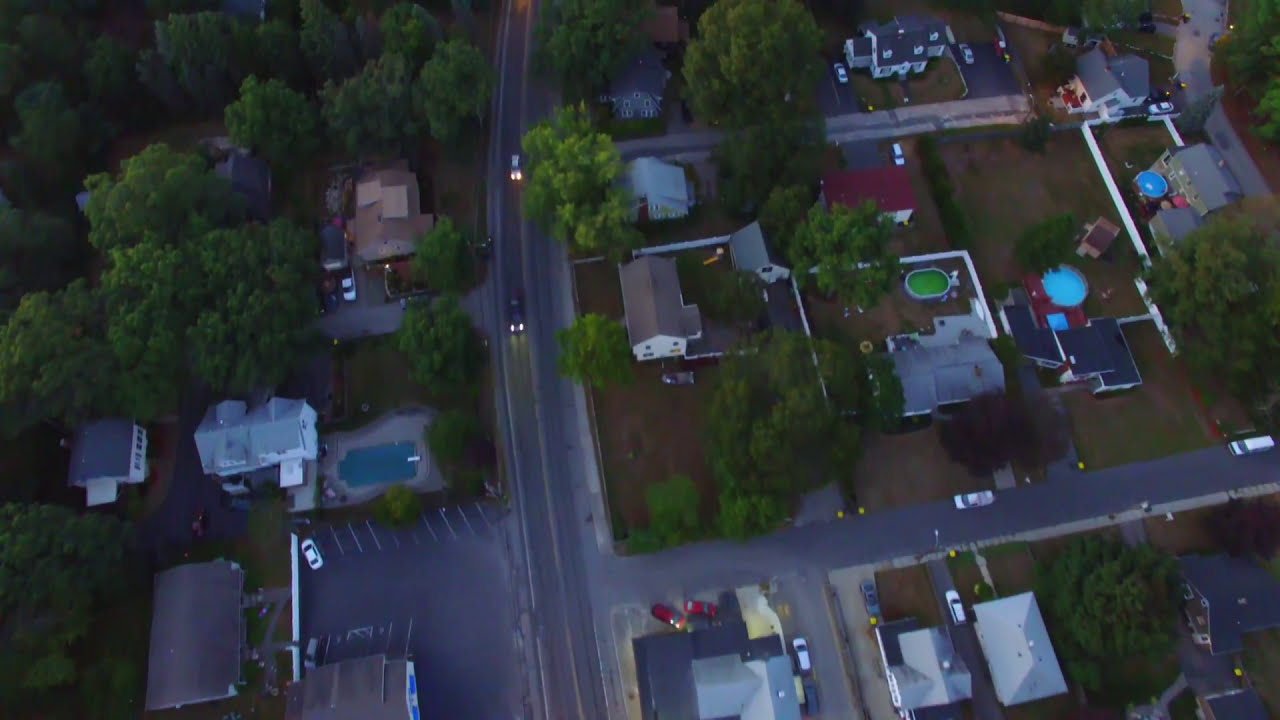The image is an overhead, possibly drone-captured, view of a mixed residential and business area at dusk, illuminated by the headlights of various cars. The main road runs vertically through the picture from top to bottom, bordered by two traveling cars with headlights switched on. This road curves left at the bottom into a parking lot, where a white car can be seen, and branches off right into another road lined with parked cars.

On the left side of the picture, the upper-mid to upper-left region is dense with bushy, not particularly tall, green trees. Various buildings populate this area, including a brown building, a white one, and a smaller white building with a black roof. Towards the bottom-left, there’s another small structure with a black roof.

In the central and right segments of the image, a patchwork of buildings is visible, including houses with distinctive roofing: a brown-roofed house, a light green-roofed house, and a darker-colored house partially obscured by trees in the upper part of the image. A prominent house with a black roof and white paint, situated mid-right, features a pool with a brown patio area behind it. Beneath the road that branches to the right are additional homes, mainly with white roofs, several housing parked white cars.

The image showcases several red cars scattered throughout, and most notable of the vehicles, apart from the ones moving on the main street, include those parked on the side roads and within parking lots. The area exhibits more brown soil with sparse green patches rather than lush grass, emphasizing a somewhat arid appearance. The overall scene is subtly dimmed, suggesting the approach of evening.